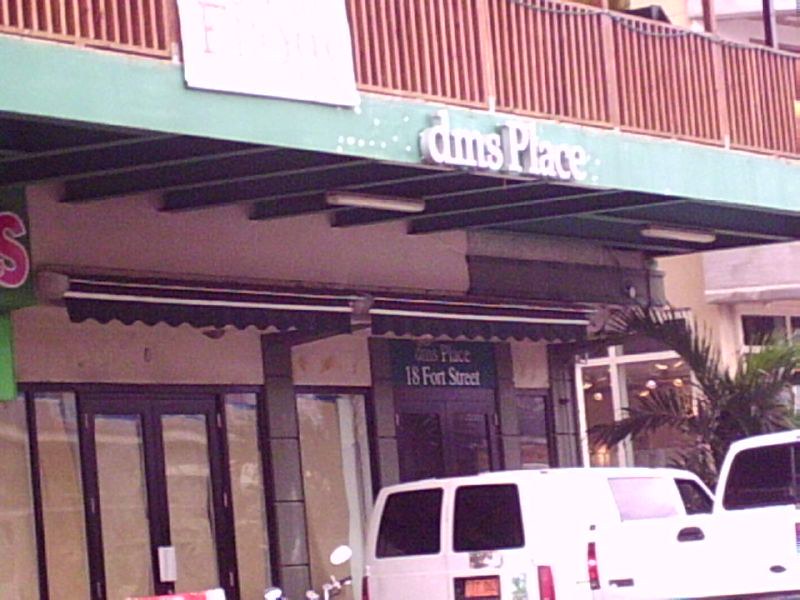This image captures the exterior of a two-story building, possibly a storefront or restaurant, located at 18 4th Street. The photo appears to be taken from a parking lot or street, as indicated by the presence of a white pickup truck, a white van, and the handlebar of a motorcycle partially visible in the foreground. The building features an entry door and several windows that are obscured by what seems to be white paper. Prominently displayed above the entrance is a green sign that reads "DM's Place". In addition, a second sign with the same lettering is visible on the rust-red railing of a balcony on the upper floor.